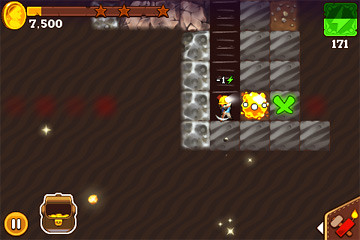This screenshot is from a 2D video game, likely a mobile or older game, with a theme rooted in mining gameplay. The central character, dressed in blue with flame-like hair, is navigating a grid composed of cubes, each portraying different textures such as boulders, rock, and what looks like a ladder. Notably, one cube features a glowing green 'X,' while another depicts an explosion. Surrounding these, a yellow creature and what seems to be a miner’s helmet in yellow can be seen. The background exhibits black and gray wavy lines accented occasionally by gold or yellow glowing stars. At the top of the screen, a score of 7,500 is displayed. Additionally, the interface includes images of coins and in-game currency in the top corners, a pause button and treasure chest illustration in the bottom left, and a hammer icon in the bottom right, suggesting building options.